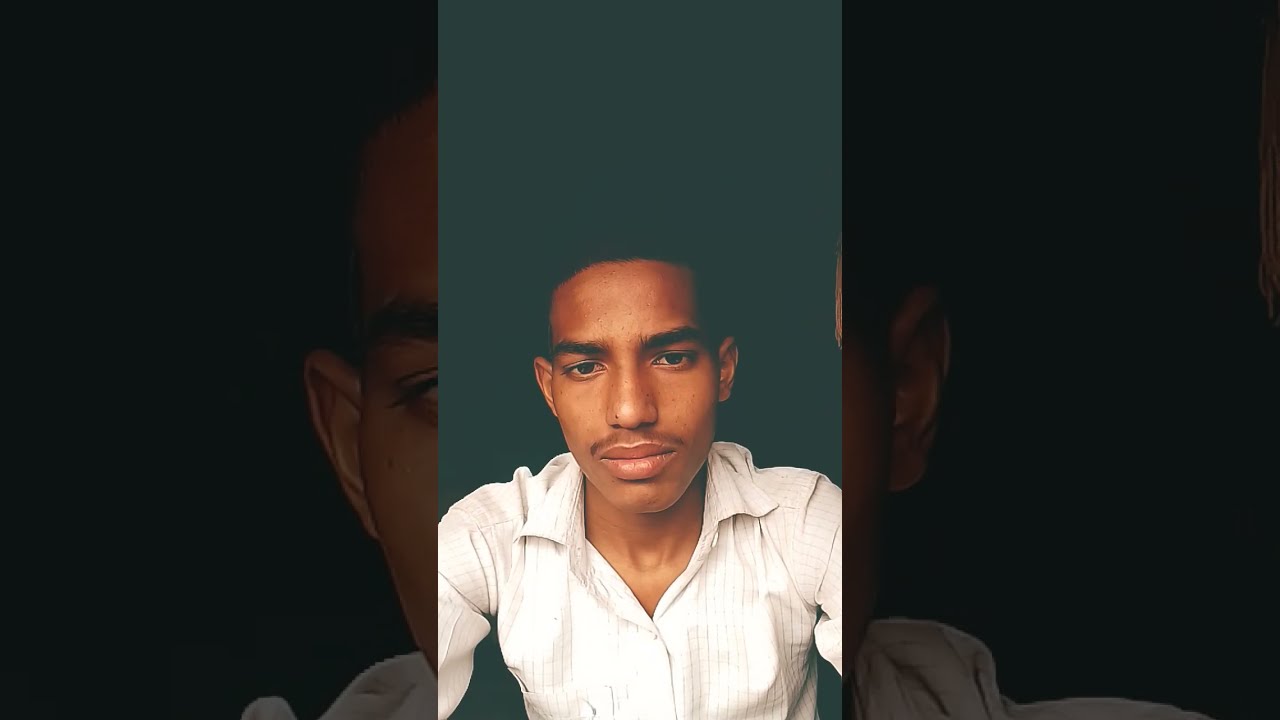The image depicts a photograph of a young black man with dark features, positioned in the bottom half of the frame. His complexion is brown, his eyebrows bushy and dark, his eyes intense, and his lips full and pink. He has a small moustache, no beard, and a broad nose. The man is gazing slightly below the camera with a contemplative, serious expression is solemn, adding a sense of gravity to the image. His dark hair blends seamlessly into the dark grey background, making it almost indistinguishable. He is dressed in a white collared button-down shirt with a subtle grid-like texture. The photograph is the focal point of the composition, dividing the image into three vertical sections. The left and right sections are darkened, blurred close-ups of his face from the middle section, emphasizing the central portrait. The overall shape and size of the image resemble a high-definition television screen.